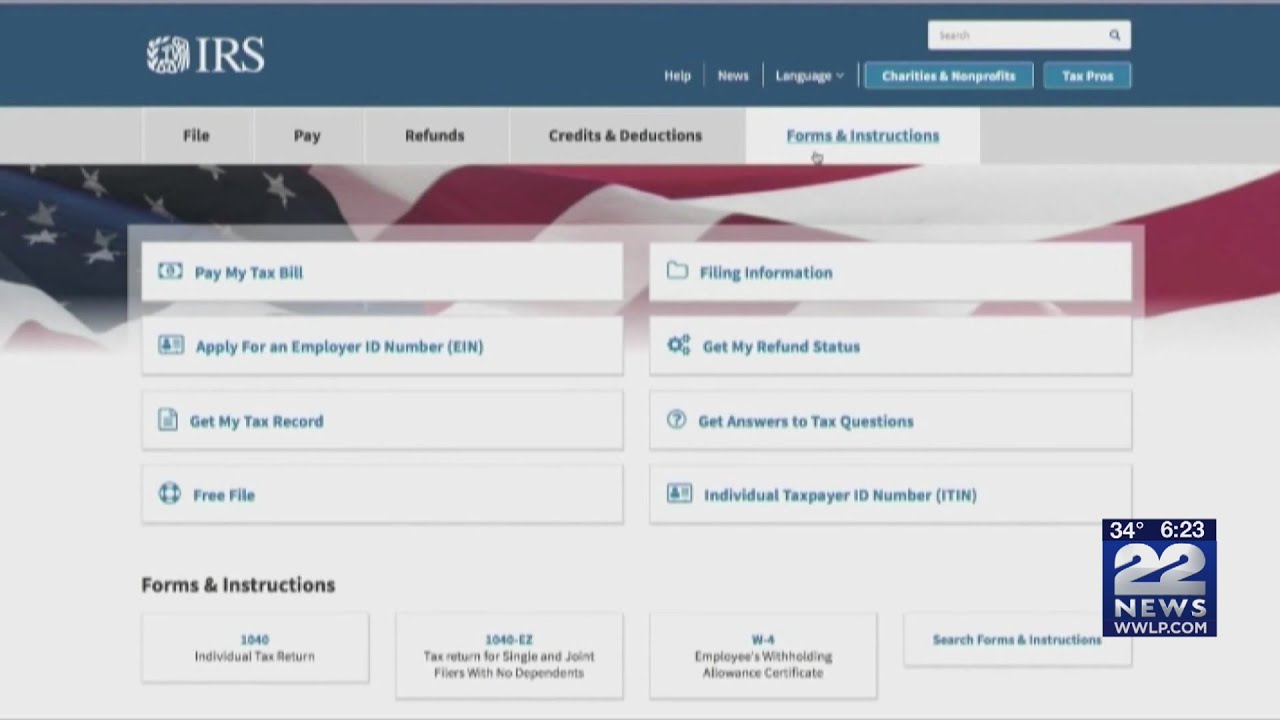The image depicts the official webpage for the IRS. At the top, the header features a navy blue background, with the IRS logo positioned towards the left. The logo consists of a white balance scale of justice in the center, flanked by several leaves curving towards the right, and what appears to be an angel wing to the right of the balance scale. To the right of the logo, the acronym "IRS" is displayed in bold, capital letters.

To the far right of the header, there's a menu with options such as "Help," "News," and "Language," each separated by thin white lines. The "Language" option includes a downward-pointing arrow to indicate a submenu. Additionally, the header features a rectangular button with a lighter navy blue background and a white border, containing bold white text that reads "Charities & Nonprofits." Adjacent to this button is another similarly styled button labeled "Tax Pros." Above all these elements lies a search bar with a white background and gray text that says "Search." A bold gray magnifying glass icon is prominently displayed on the far right of the search bar.

Below the header, the interface transitions into a light gray main menu area, where each menu option is divided by a white line and written in bold black or dark gray text. The options listed are "File," "Pay," "Refunds," "Credits & Deductions," and "Forms & Instructions." The selected option, "Forms & Instructions," is highlighted with blue text against a white background, and a hand cursor is visible to indicate this selection.

Central to the webpage is an area featuring a flowing American flag that fades into gray towards the upper center and bottom of the image, creating a backdrop for the content that follows.